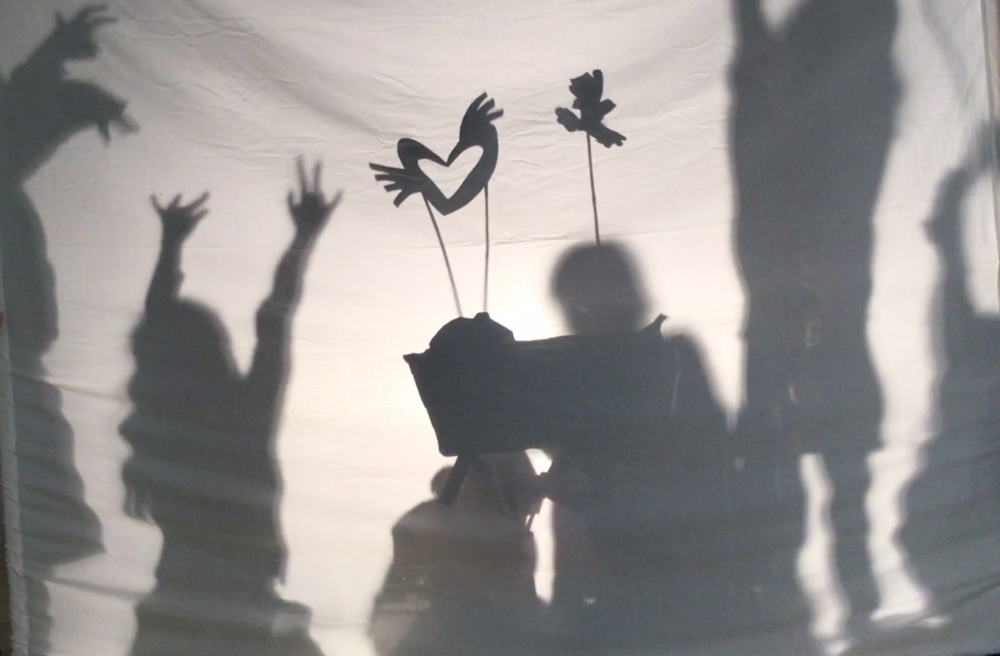The image depicts a shadow puppet show viewed from the audience’s perspective through a white sheet. Silhouettes of at least six people can be seen behind the sheet, actively engaging in the performance. On the left, two individuals have their hands raised, with one of them possibly bending down slightly. In the middle, two performers are using various props to enhance their shadow shapes, creating intricate forms like two birds or swans with their beaks and necks intertwined to form a heart shape, supported by visible strings or sticks. Additionally, there's an item resembling a boat, seemingly floating with a hat attached to it, which might be shaped by someone's hand. On the right side, another two people stand with their hands raised, and one appears to be jumping, adding a dynamic element to the scene. Overall, the meticulously crafted shadows and props create a captivating and intricate visual story on the white canvas.